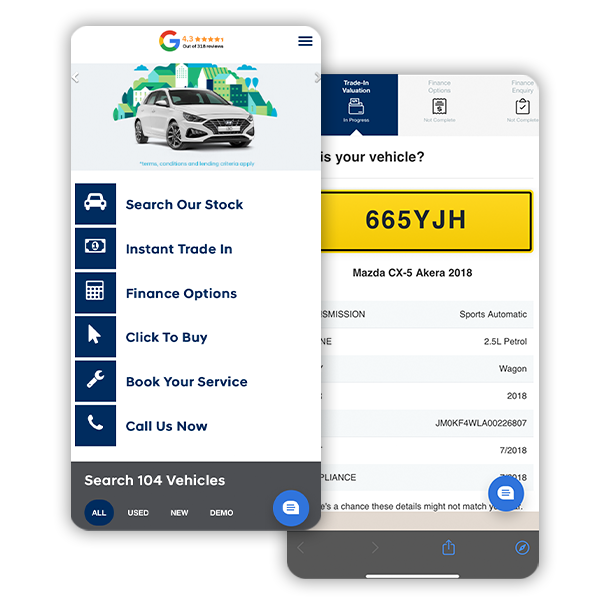The image displays two screens from a mobile phone showcasing a car dealership's app interface. At the top, the app is branded with "Google" and is rated 4.3 stars out of 5. A white car with grayish tones, illustrated against a backdrop of buildings and greenery, occupies a central position. 

Key features on the first screen include options labeled "Search Our Stock," "Instant Trade-In," "Finance Options," "Click to Buy," "Book Your Service," and "Call Us Now," all presented in blue text on a white background accompanied by respective icons. The bottom of this screen features a dark gray section with text indicating "Search 104 Vehicles" in white, alongside a blue 'All' button, and options for "Used," "New," and "Demo" categories. A chat feature is visible on the lower right corner.

The second screen highlights a specific vehicle detail. It mentions "Your Vehicle" at the top, adorned with a gold box containing the text "665YJH" in blue. Below, it lists a Mazda CX-5, describing it as a sports automatic petrol wagon from 2018. Partial information, including a VIN number ending in "7218," is visible, though some details are cut off. This screen also features a chat option.